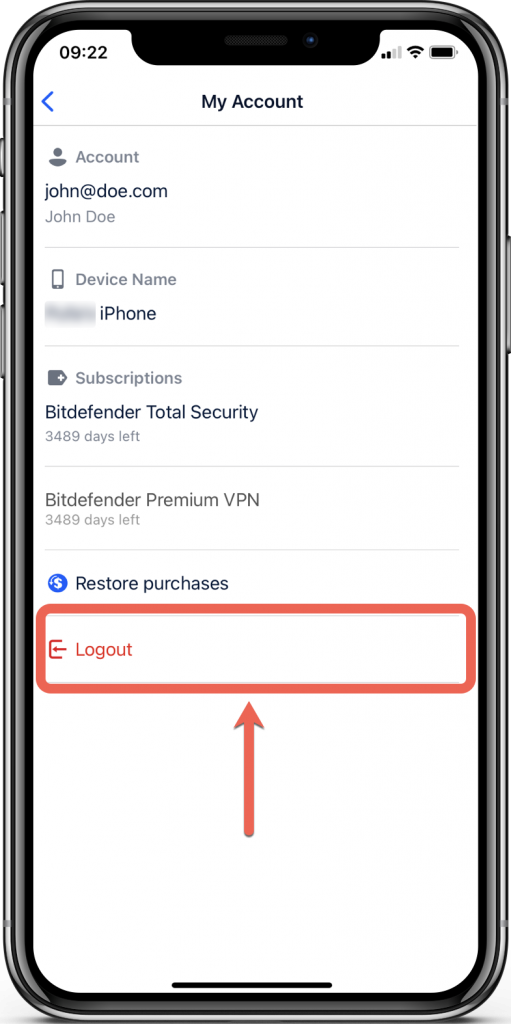**Detailed Image Caption:**

This image captures a phone screen with a dark gray rim. At the top center of the phone is a front-facing camera lens. The screen displays several details and icons:

- **Top Bar:**
  - Top left: The time is displayed as 09:22 (9:22 AM).
  - Top right: Indicators show a cell phone signal with two out of four bars, a WiFi connection symbol, and a nearly full battery icon.

- **Main Screen:**
  - Centered at the top in black text: "My Account".
  - Top left: A blue back arrow.
  - Below "My Account", there is a horizontal gray line break.

- **Account Section:**
  - Left: A round person icon in gray.
  - Right of the icon: "Account" in gray.
  - Below this, in black text: "john@doe.com".
  - Underneath "john@doe.com", in gray text: "John Doe".
  - Another horizontal gray line break follows.

- **Device Section:**
  - Left: A small cell phone icon.
  - Right of the icon: "Device Name" in gray.
  - Below this section is a blurred out text area to the left with "iPhone" to its right.
  - Following this is yet another horizontal gray line break.

- **Subscriptions Section:**
  - Left: A gray tag symbol with a plus (+) sign.
  - Right of the symbol: "Subscriptions" in gray.
  - Below this, in black text: "Bitdefender Total Security".
  - Underneath: "3,489 days left" in gray.
  - Below these details, another horizontal gray line break.
  - Following is "Bitdefender Premium VPN" with "3,489 days left" below it in gray text.
  - Yet another horizontal gray line break follows.

- **Restore Purchases Section:**
  - Left: A blue round icon with a white "S".
  - Right of the icon: "Restore Purchases" in black text.
  - Below this, there is a prominent rectangular box outlined in red.
  - Inside the red box, on the center left side: A left-pointing arrow with the label "Log Out" written in red.
  - Below the box, an arrow points vertically up to highlight the "Log Out" feature.

- **Bottom Center:**
  - A small black horizontal line indicating a scrolling element, suggesting a tab or navigation option.

The meticulous arrangement of elements and clear use of icons are presumably designed for easy navigation within the account management interface.